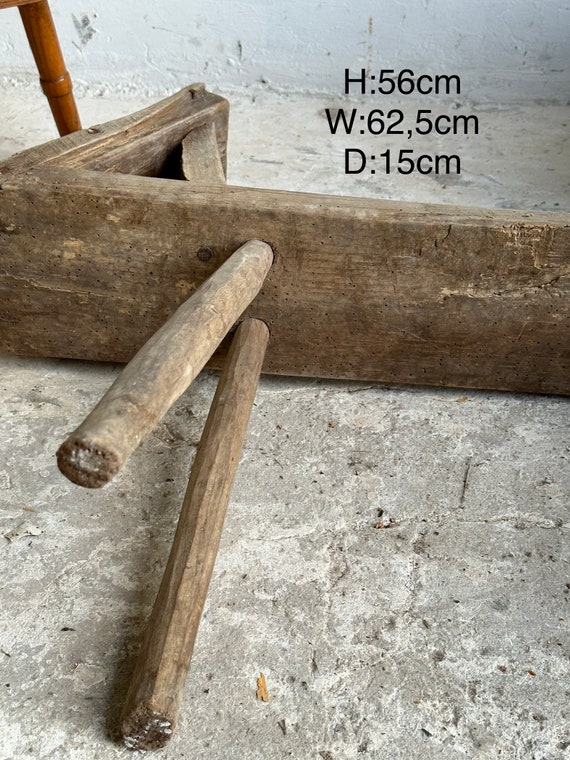The image depicts an old, roughly constructed wooden piece lying on its side on a light gray, cracked stone surface with a marbled texture. The wood appears aged and rotted, displaying a light brown color and uneven texture with visible nails. It features two uneven wooden dowels sticking out from the bottom, pointing towards the camera. The structure seems to resemble a carpentry piece, although its exact purpose is unclear. In the background, there's a leg of a chair, though the rest of the chair is not visible. The image is accompanied by text indicating the dimensions: a height of 56 centimeters, a width of 62.5 centimeters, and a depth of 15 centimeters. The setting appears to be indoors, with light-colored walls in the background.